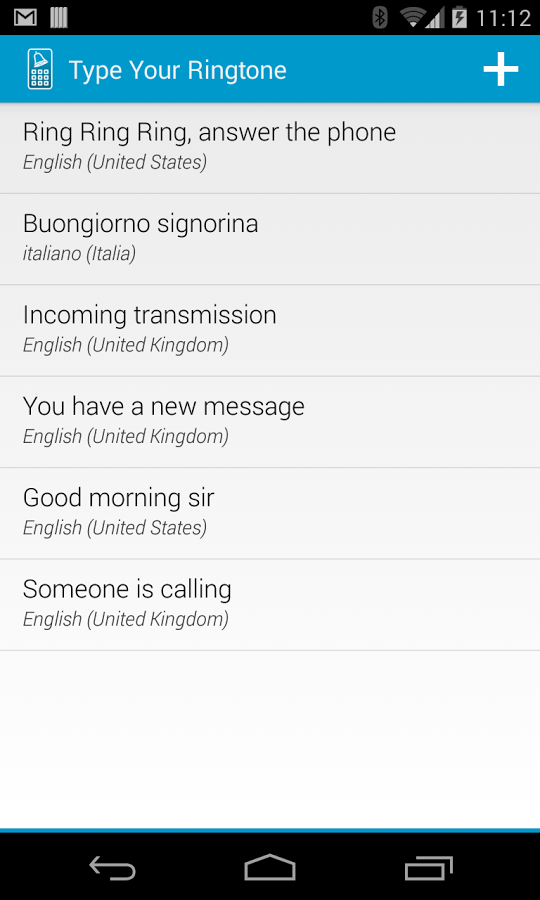A rectangular smartphone display shows several rows of application icons. The icons for Gmail and Bluetooth are clearly visible, indicating available email services and Bluetooth connectivity. Notifications for messages and incoming calls are displayed, with phrases in multiple languages including English, Italian, and specific mentions of the United States and the United Kingdom. The screen also shows an incoming transmission alert with a greeting in Italian: "Buongiorno, signora," and details in English such as "Good morning sir" and "Someone is calling." 

Instructions for customization options like setting a ringtone ("Type your ringtone") and visual indicators such as arrows pointing left are also present. The display appears organized in 123456 rows, featuring text and icons related to communication and notification features. Touch interaction prompts like "Touch the part" suggest a user-friendly interface designed for easy navigation through various alerts, settings, and notifications.